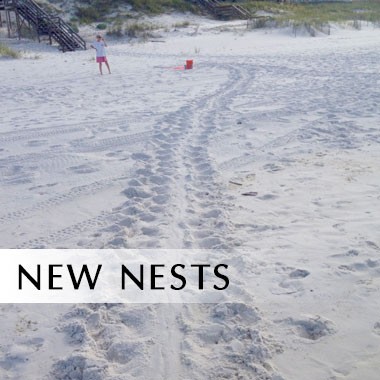The image depicts a snowy or sandy beach with a prominent set of tracks running diagonally across the foreground, suggesting the passage of a vehicle but not definitively identifiable as tire tracks. The tracks are accompanied by numerous human footprints, adding texture to the scene. In the upper right-hand corner of the image, dark stairs lead away from the beach, contributing to the depth and context of the setting. A young man wearing a white t-shirt and red shorts stands in the middle distance, slightly off to the left. Approximately six to eight feet to his right is a red bucket. The background features some sparse greenery. In the lower left-hand corner, bold black uppercase letters spell out "New Nests" on a white background, suggesting the image might be an album cover.